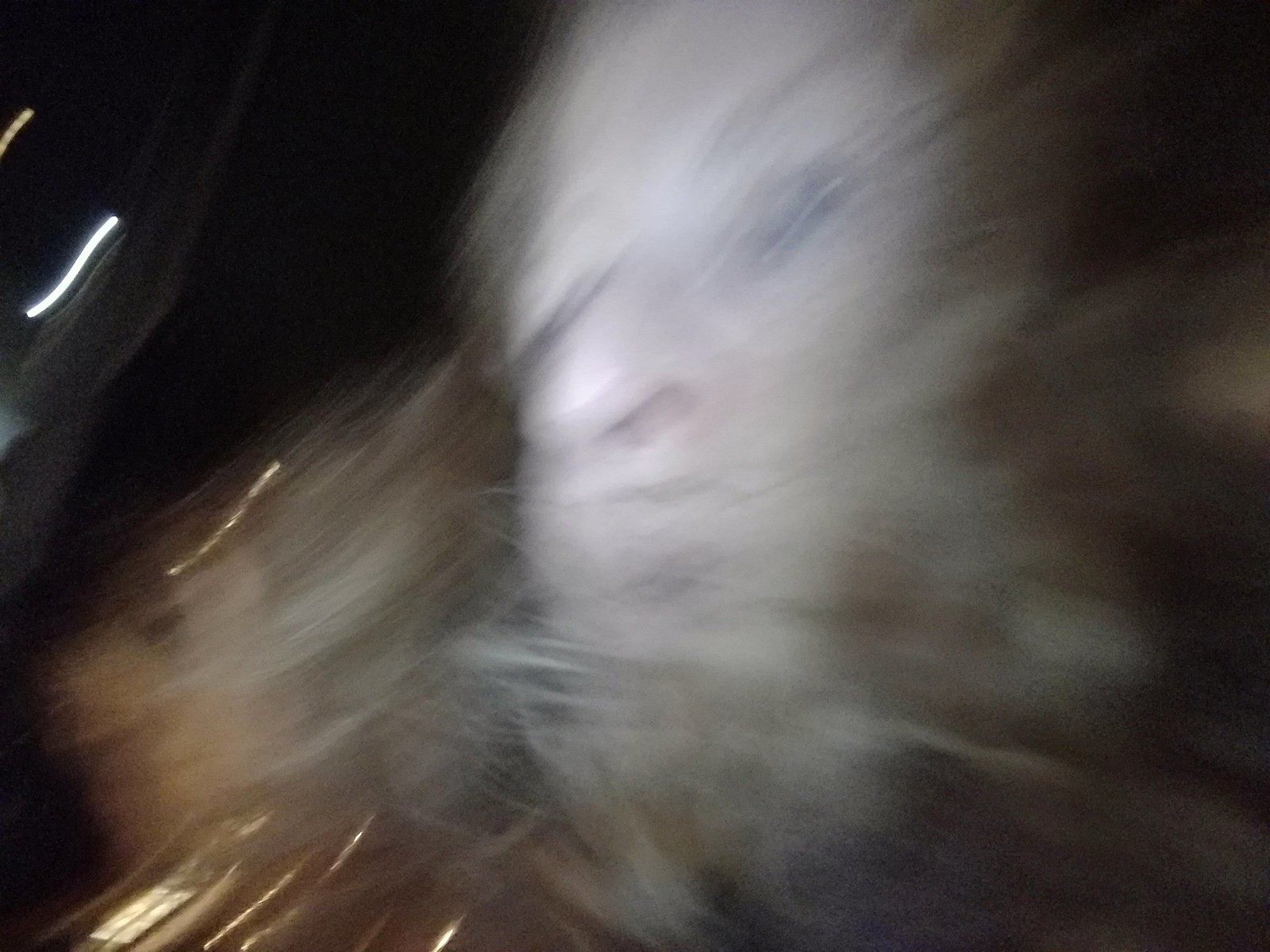In this image, an indistinct scene unfurls with a rich tapestry of colors and movement. The backdrop is predominantly jet black, adding an element of mystery and depth. To the left, a set of white and yellow light stripes slices through the darkness, illuminating the immediate area with a touch of gray. At the bottom left corner, a splash of yellow light further punctuates the scene.

At the forefront, a person's face emerges – or rather, the suggestion of it. The light tan hues and streaks of brown suggest hair in motion, blurring and partially concealing the facial features. Despite this, the lines of the eyebrows, the vague shapes of the eyes, and the nose can still be traced. The image’s blurriness adds a dynamic, almost ethereal quality, capturing a fleeting moment in time. The photograph resonates with an intriguing, almost chaotic beauty.